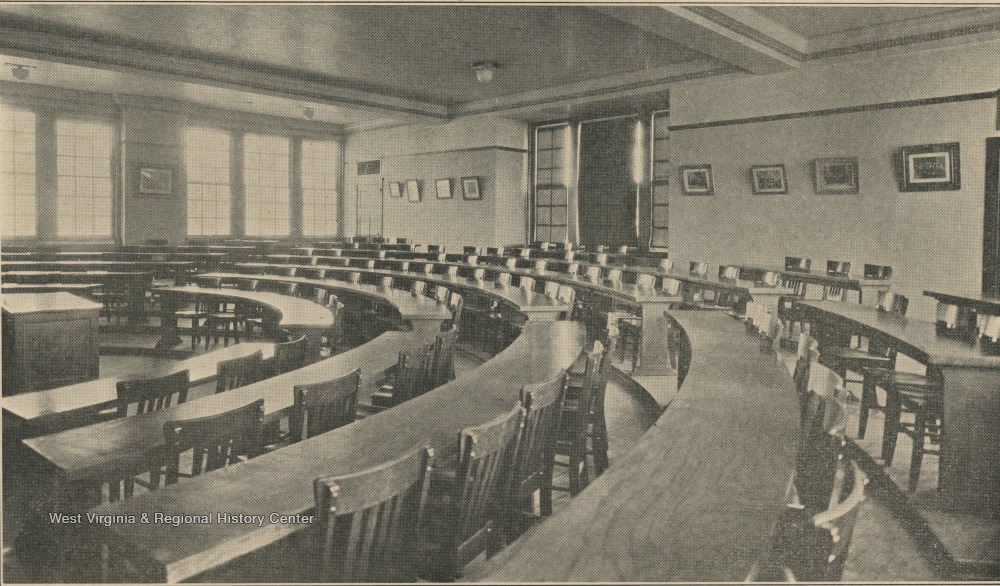This monochrome image, likely from the 1800s or early 1900s, depicts a vintage, empty university lecture hall. The hall features a wooden podium situated to the extreme left of the image. Surrounding the podium are multiple rows of curved, long, wooden tables with straight-backed wooden chairs, arranged in a semi-circular pattern. The tables grow in size as they radiate outward, forming a large arc across the room. There are walkways between the rows, segmenting them into distinct sections. Visible on the back wall are eight framed photographs, and to the left, there are five tall, paned windows allowing sunlight to stream into the room. A doorway is also seen at the back right. The lower-left corner of the photograph bears the text "West Virginia and Regional History Center."